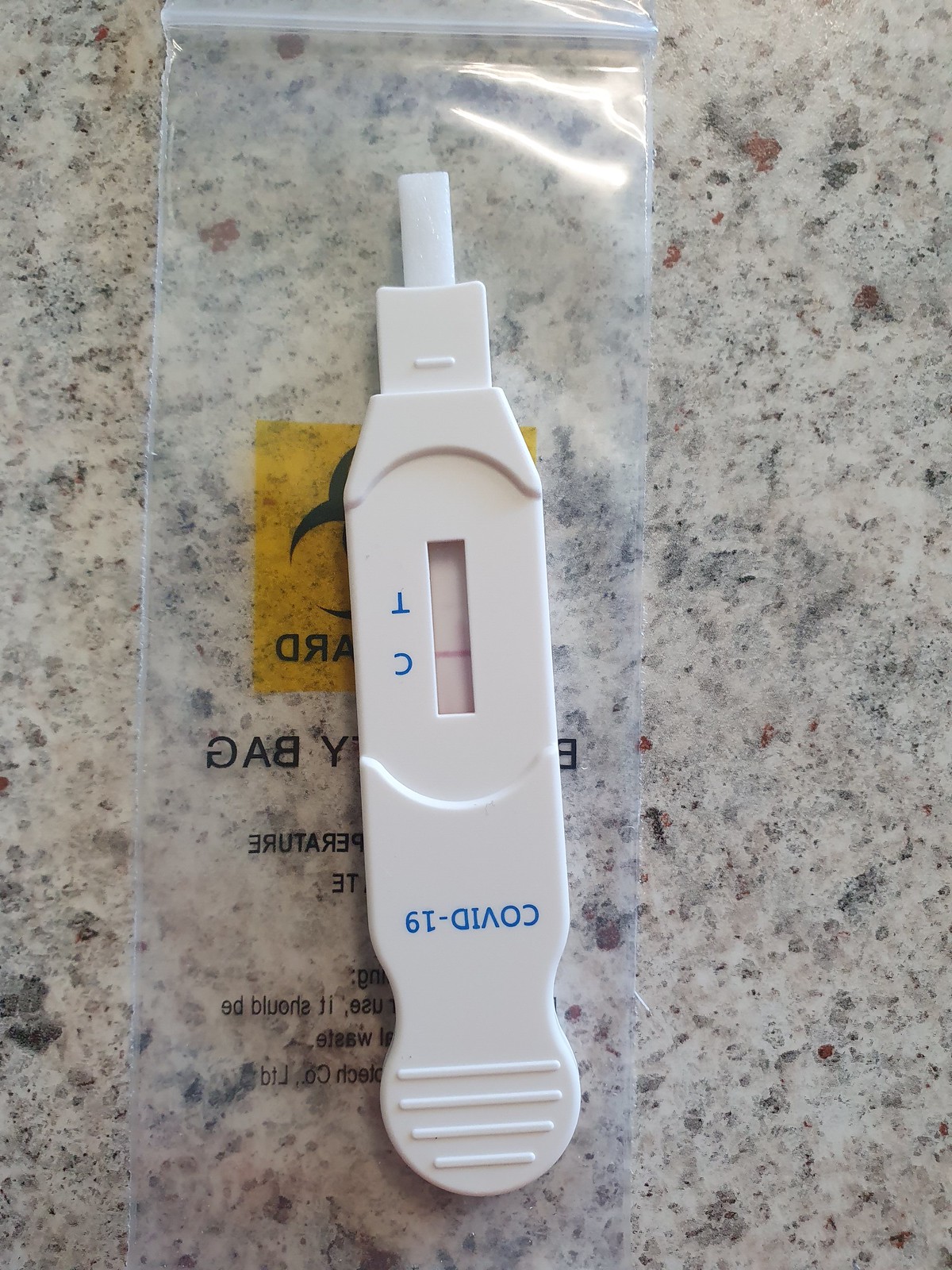In this photograph, a COVID-19 rapid antigen test kit is prominently displayed on a granite surface characterized by its beautiful grayish color with flecks of darker gray. The white, oblong test strip is positioned upside down, rendering the text "COVID-19" readable but inverted. An insert window on the test strip appears pinkish, and the upside-down letters "CT" are visible within it. The tip of the test strip rests on a very narrow Ziploc bag, which bears some partially obscured, backward-written text. Additionally, a small section of a logo is visible on the bag, consisting of a yellow square with a black graphic and a few indecipherable letters.